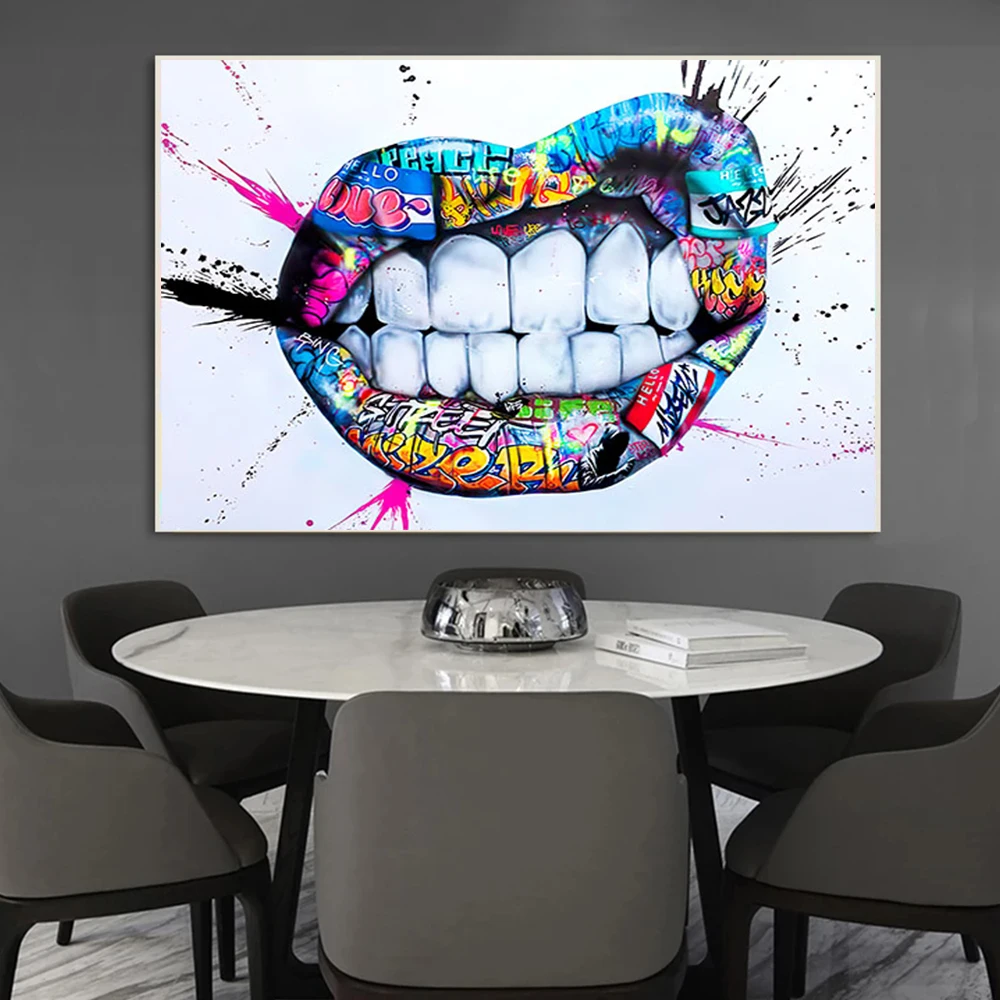This photograph captures a room that appears to be part of an office building, possibly a conference or break room. The room features a medium gray wall and a stone-like floor, likely a marble or granite cover. At the center, there is a round, white, marble-looking table surrounded by six dark gray upholstered chairs, all with black tubular legs arranged neatly around it. Atop the table rests a shiny silver decorative bowl and two white books.

The main focal point of the room is a large, rectangular piece of modern art hanging on the gray wall above the table. This striking artwork features a close-up of a human mouth with giant white teeth. The lips are vividly graffitied in an array of colors including blue, fuchsia pink, teal, red, yellow, orange, and green. These colors also seem to splash onto the white matte background. Several name-tag stickers are visible on the artwork, one with the word "Jazz," another saying "Hello," and yet another with "Love." The bold colors and modern style of the artwork create a stark contrast to the otherwise neutral-toned and formally arranged room.